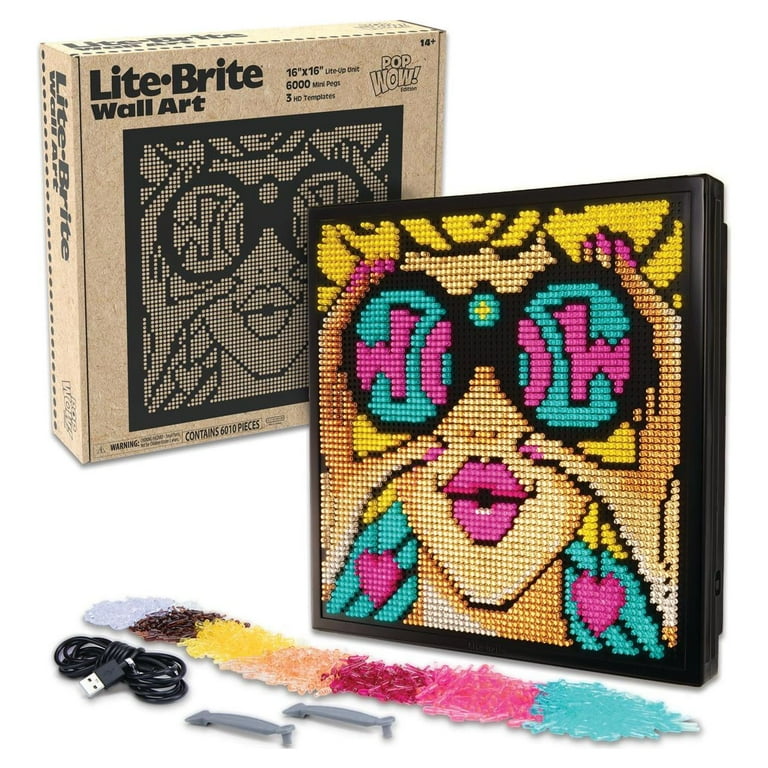This image showcases a detailed product listing for an arts and crafts kit designed to create light-up wall art. The kit, branded as "Lite-Brite Wall Art," is packaged in a brown box, prominently featured on the left side of the image. The packaging displays the product name "Lite-Brite," with "wall art" and dimensions "16 by 16" inches noted beneath it. The kit includes 6,000 mini pegs and 3 HD templates. Inside the box, users can create vibrant art, such as the highlighted example of a pop-art style face of a blonde woman with yellow hair, pink earrings, and bright pink lipstick. The woman is depicted holding binoculars that spell out the word "WOW" in bold pink letters. The image also displays the vivid color pegs used, including white, brown, yellow, orange, red, pink, and blue. Additionally, a USB cord is featured, indicating the artwork lights up when connected.